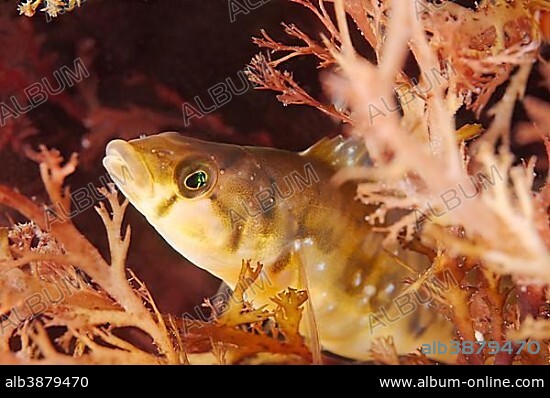This underwater scene showcases a tropical fish, resembling a small gunnel or a sea bass, amidst vibrant plant life. The fish, characterized by its dirty mustard yellow-green color and speckled spots along its back, is prominently positioned in the center of the image. Its body extends diagonally from the lower right corner to the upper left corner, displaying its side profile and keen eyes. Surrounding the fish is a lively array of sea plants, predominantly in shades of orange, pink, and red. The lower part of the image features a black band with partial text "ALB3879470" and a URL "www.album-online.com." Additionally, there are multiple hazy white "album" watermarks scattered throughout the image, contributing to its stock photo nature.